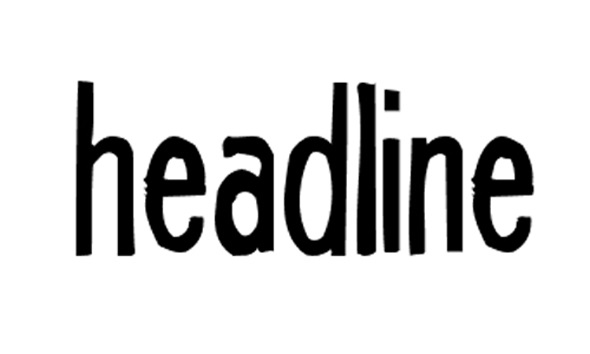The image displays the word "headline" in black, lowercase, printed font prominently in the center against a plain white background. The text appears hand-drawn, possibly with a thick black marker or Sharpie, giving it a slightly varied and jagged appearance, particularly on the left side of the two 'E' letters. The font is not fancy or cursive, but rather a basic, condensed typeface that adds a raw, informal touch to the otherwise straightforward word presented. The uneven thickness of the letter strokes and minor irregularities within, especially on the semicircle parts of the 'E's, contribute to its imperfect yet distinctive look, suggesting a more casual or handmade style.